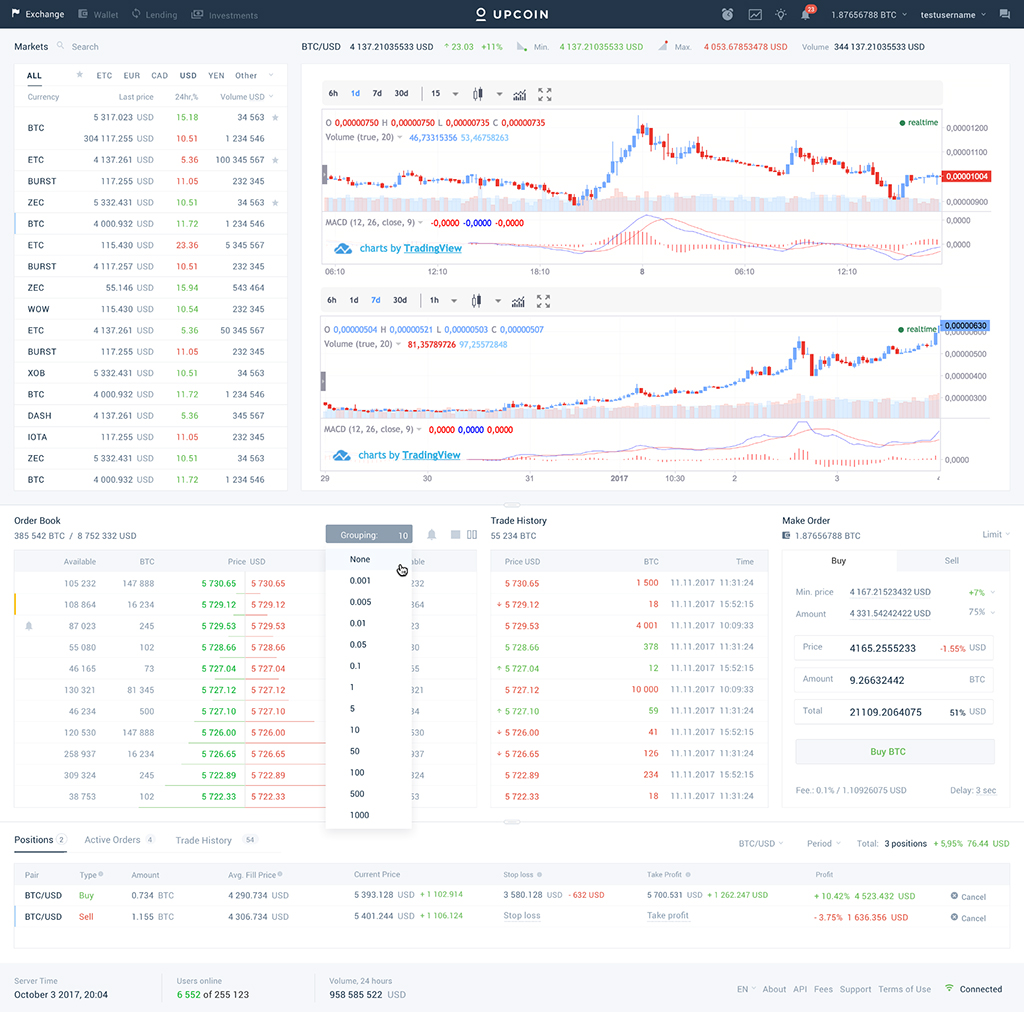In this image, we see a detailed interface of a platform called Upcoin. At the very top of the interface, there is a narrow, rectangular, horizontal section with a black background. This top section features four categories on the left, the "Upcoin" logo in the center, and a few icons on the top right.

On the main page, starting from the top left corner, we observe the name of a coin along with three separate sets of data positioned to its right. Towards the right side, there are three distinct line graph charts displaying data in either red or blue text, each chart varying in data representation.

Proceeding downwards, the next section includes three separate areas of information. On the left, labeled "Order Risk," the middle section is titled "Trade History," and the right section is named "Main Order." Each of these sections contains charts filled with numerical data and corresponding categories.

At the very bottom of the interface, there are three sections on the left side with black text, and two additional sections located on the bottom right, showcasing even more data.

Overall, the image encapsulates various data points and informational charts, designed to give a comprehensive overview of cryptocurrency data on the Upcoin platform.